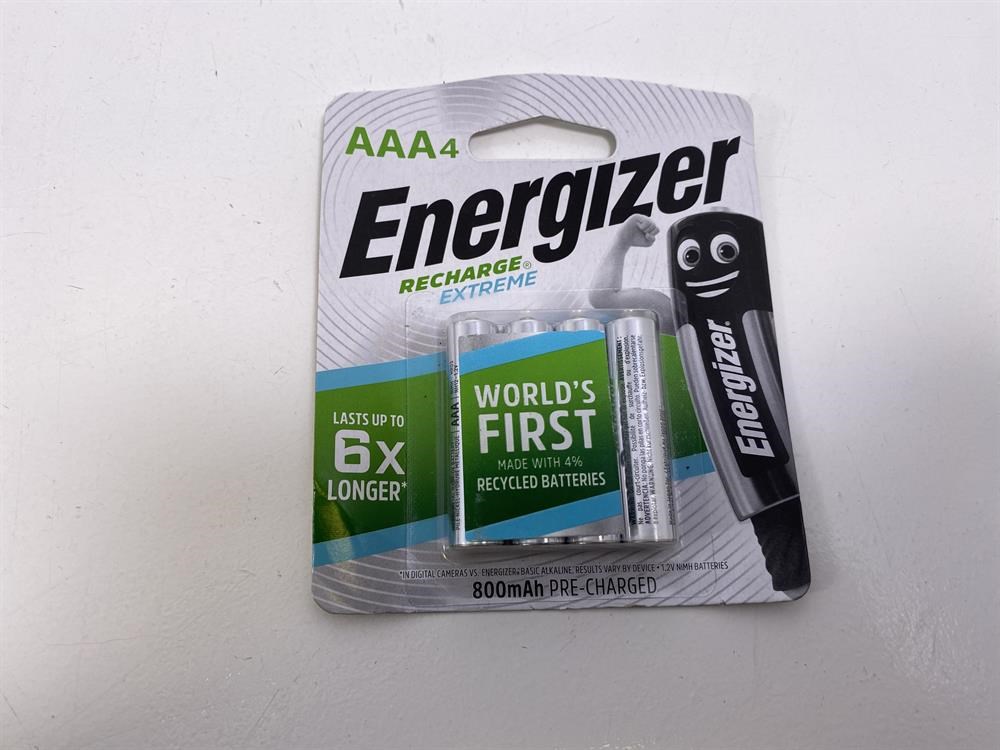The image displays a pack of Energizer Xtreme batteries, specifically featuring four AA batteries encased in a clear blister pack. The packaging rests against a white background, with a gray shadow stretching diagonally from the bottom left-hand corner to the lower right-hand corner. The blister pack is backed by a cardboard insert designed with radiating concentric circles.

Prominently, the package design starts with "AAA" in lime green letters, followed by the number "4" in slightly smaller font. The brand name "Energizer" is written diagonally across the package in large, bold black letters. Beneath it, "Recharge®" is boldly printed in green, and "Xtreme" is detailed in blue underneath. A smiling battery character with big, round eyes is flexing a muscle on the right-hand side of the packaging; "Energizer" is marked vertically along his body.

The batteries themselves are centered within the clear blister pack, while the left-hand side of the packaging proclaims, "Lasts up to 6x longer." A prominent banner across the batteries highlights "World's First made with 4% recycled batteries," with this section featuring a blue band on the top and bottom edges and a green center.